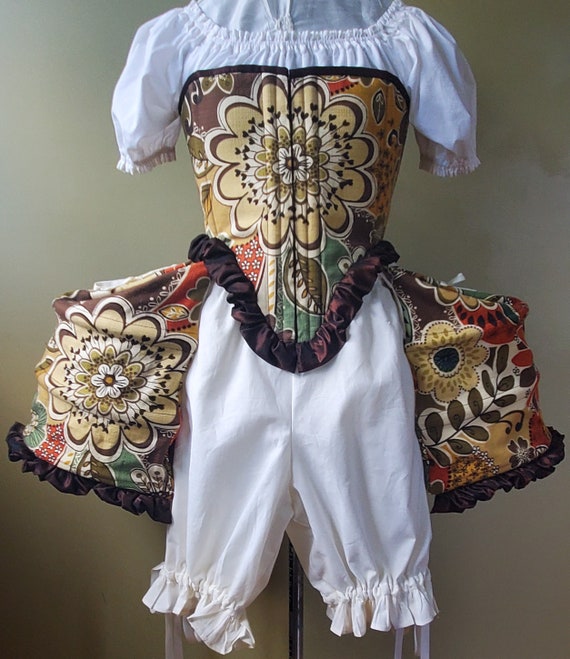The image shows a vintage, full-body dress hanging on a rack or mannequin. The dress is predominantly white with an intricate floral pattern covering the skirt and chest area. Prominently displayed in the center of the chest is a large, multi-colored flower with hues of yellow, white, brown, red, and green. This flower is surrounded by smaller floral designs that extend concentrically outward, showcasing a complex blend of plant motifs. The chest area is further adorned with purple velvet frills at the bottom.

The dress features short white sleeves and continues the floral pattern along the torso down to the groin area. The skirt and pants of the dress include similar floral elements, with matching flowers on the skirt's left side and the chest. The pants are styled in a balloon, pantaloon fashion, tapering off with lacy or frilled edges at the knees, and adorned with a couple of strings. The design reflects historical fashion, potentially from the Middle East, emphasizing an elaborate and decorative aesthetic.